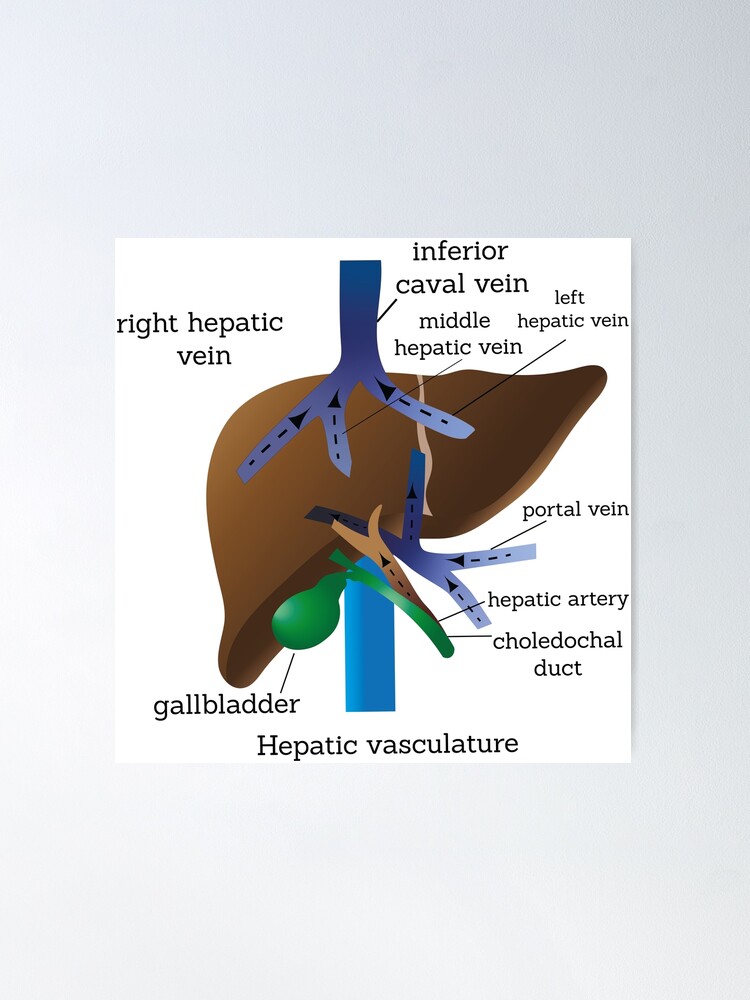This detailed medical illustration depicts the liver and gallbladder anatomy, set against a light gray background with a white box and light drop shadow. In the center, the large brown liver is the main focus, shaped somewhat like a shoe. Emanating from the liver, several key structures are labeled. 

Starting from the left, the right hepatic vein is identified, followed by the blue inferior caval vein that branches into the liver. The middle and left hepatic veins are also labeled within this blue network. At the bottom left of the liver, a green balloon-like structure labeled as the gallbladder connects to the liver. Adjacent to the gallbladder, the bile duct (choledochal duct) extends towards the bottom right. Above the gallbladder, the hepatic artery and portal vein are illustrated, also connecting to the liver. 

Finally, at the bottom of this detailed diagram, text reads "Hepatic Vasculature," emphasizing the depicted network of veins and arteries integral to liver function.